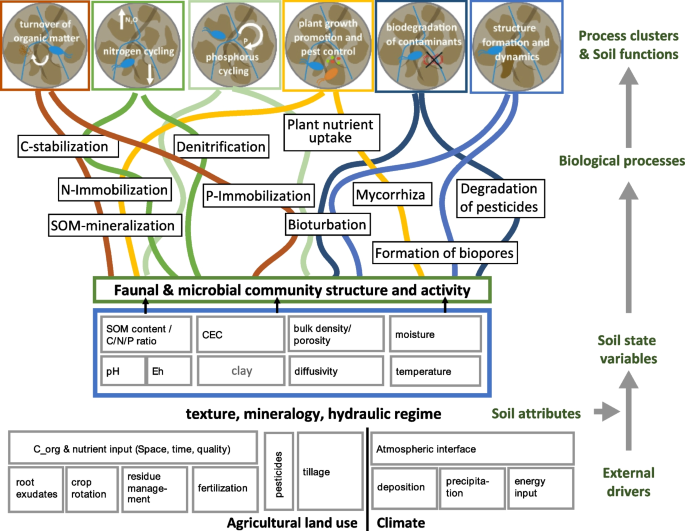The image is a comprehensive scientific diagram likely aimed at farmers, illustrating the complex interactions within an agricultural ecosystem. At the top, there are six outlined squares, each with different colors—one red, two green, one yellow, and two blue—containing circles of brownish color. Each square is labeled with scientific terms such as "Turnover of Organic Matter," "Nitrogen Cycling," "Phosphorus Cycling," and "Structure Formation and Dynamics." These squares are interconnected by arrows matching the color of their respective boxes.

For instance, arrows emanating from the yellow square, which addresses topics like "Plant Growth, Formation, and Pest Control," lead to other labeled boxes such as "Plant Nutrient Uptake," "P Immobilization," and "Formation of Bio Pores." Ultimately, all these arrows converge towards a central green square labeled "Faunal and Microbial Community Structure and Activity."

Surrounding this central network are additional squares and rectangles connected by arrows, labeled with various environmental and soil factors such as "Moisture," "Energy Input," "Deposition," "SOM Content," "CEC," "Bulk Density," "Temperature," and "Diffusability." The diagram is complex, showing the flow and interdependence of agricultural and ecological processes.

At the bottom, the diagram references broader contexts like "Agricultural Land Use" and "Climate," indicating the overarching influences on the depicted interactions. This detailed layout aims to provide farmers with a visual representation of the myriad factors influencing soil health, plant growth, and overall ecosystem dynamics.